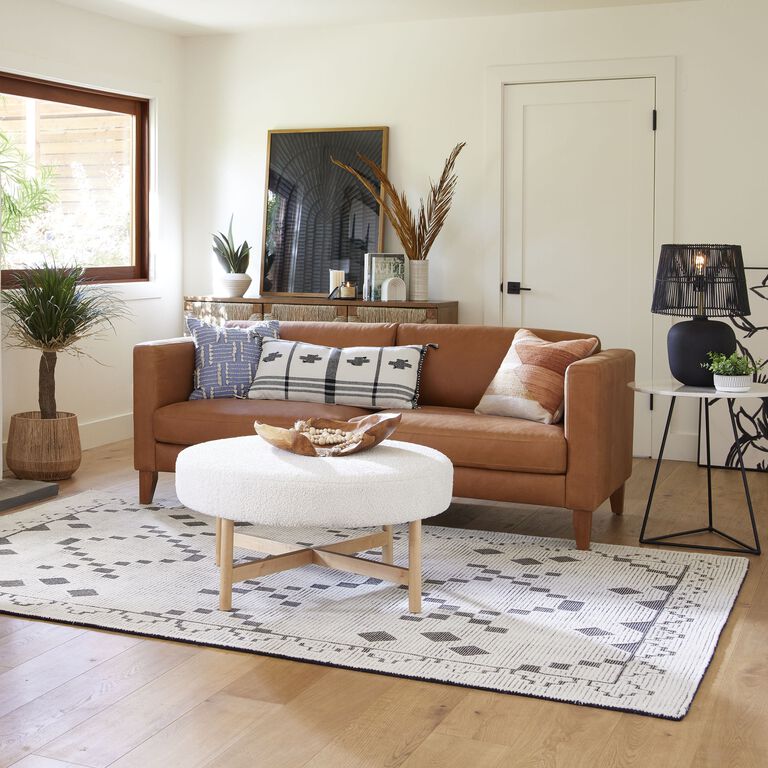This image depicts a cozy and well-decorated living room with detailed features. The centerpiece is a brown couch adorned with three pillows: a long one towards the left, a square blue and white pillow on the left side, a brown patterned pillow on the right, and a central pillow in white and gray tones. The couch partially rests on a white rug with intricate brown and black shapes, with its two front legs on the rug while the back legs are off. In front of the couch is a round footstool with wooden legs, holding an indistinct item on top. To the left of the scene, a large window with wooden brown trim reveals a view of a tree outside, with a plant below it inside the room. 

The room features white walls and hardwood floors, with a door on the right sporting a black doorknob. Placed beside the couch is a coffee table with a cushioned white top and wooden legs, holding a decorative brown plate. Adjacent to this coffee table, an iron-legged side table with a white top supports a black lamp and a small plant. There is another table in the room, characterized by black triangular legs, also housing a black lamp and a short flower. A dresser with a mirror and two plants – one tall and brown, and the other small and green – further accentuate the room's charm. The overall ambiance of the room is warm and inviting, complemented by the natural greenery both inside and outside the space.